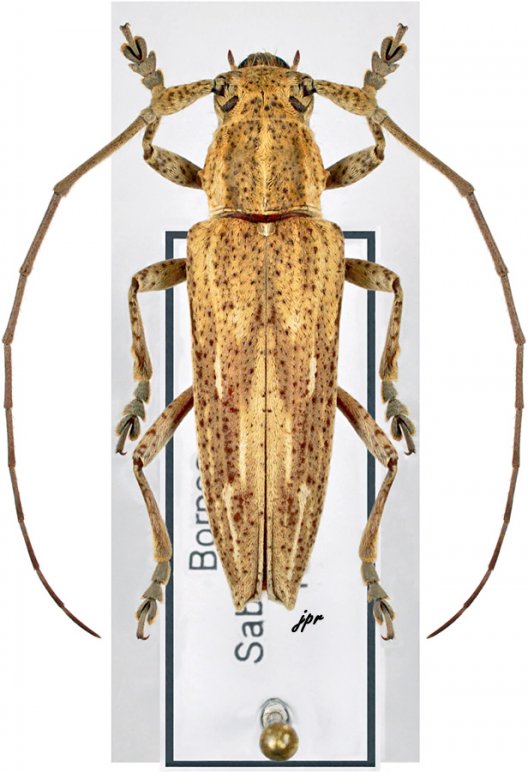A meticulously detailed image showcases a light tan, cockroach-like bug specimen with dark brown speckles, captured from a bird's eye view. The specimen features two very long antennae, extending the full length of its body, starting from near its black eyes and stretching back to its rear legs. These antennae sweep to the sides, accentuating its elongated form. The bug also possesses six legs, each ending in brown, claw-like feet. Notably, two small fangs are visible in front of its eyes, adding to its intricate appearance.

The bug is displayed atop a labeled surface, likely identifying it, with the text "JPR" written in a cursive font visible below the body. Additionally, a tack strip secures the label, suggesting a methodical presentation often seen in scientific specimen displays. The letters "BOR...SAB" also appear vertically beside the bug, partially obscured by its body.

The image looks expertly cleaned or photoshopped, with a potentially transparent background typical of a PNG file, emphasizing the bug's detailed features and the careful arrangement of the scientific label.